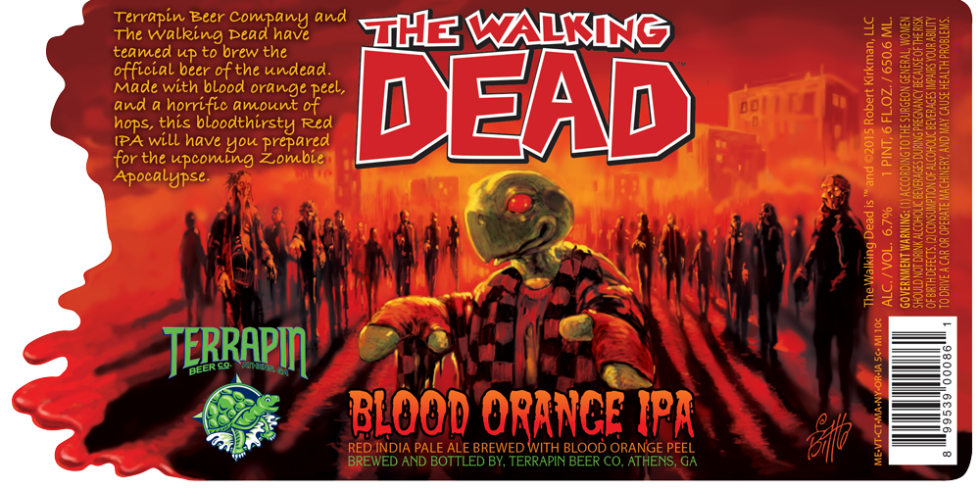The photograph showcases a beer label in a vivid landscape orientation dominated by an array of red and orange hues. The backdrop features a post-apocalyptic cityscape teeming with black silhouetted zombies. Embedded in the ominous scene is a turtle standing upright like a human, dressed in a black and red plaid shirt, red gloves, and having red eyes. Key to the label is the text “The Walking Dead” in red lettering outlined in white at the top, signifying its tie-in with the popular series. Below, in a drippy orange font outlined in black, the label reads "Blood Orange IPA." The left side features green writing with the brand name "Terrapin" alongside its logo, a turtle with a beer hops shell. The upper left corner provides a detailed description in gold lettering about the beer, declaring it the official beer of the undead, made with blood orange peel and a “horrific amount of hops,” preparing drinkers for the zombie apocalypse. Additional information can be found on the right side, including a barcode. The label effectively marries a thematic design with detailed textual elements to promote the Blood Orange IPA.